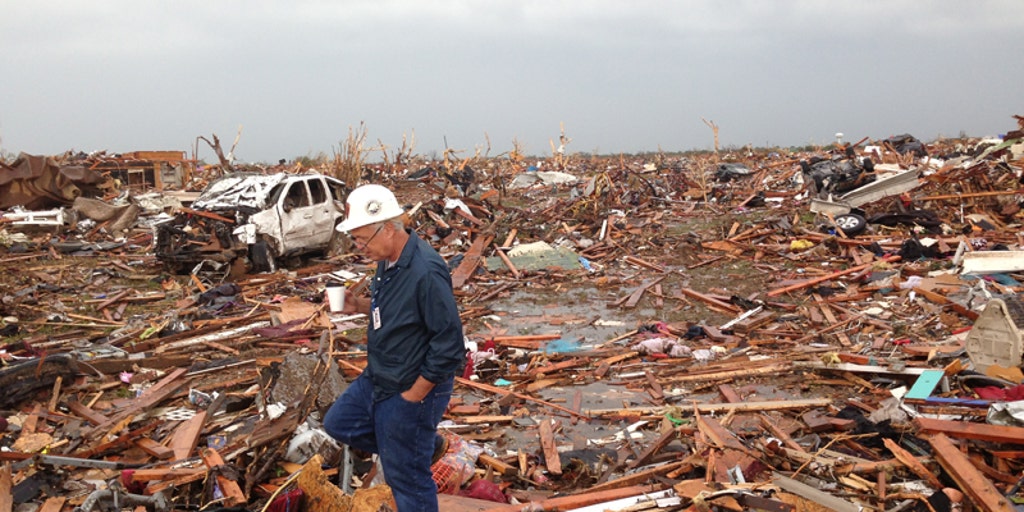This digital photograph, oriented horizontally, vividly captures the aftermath of a devastating tornado in a disaster-stricken area. The image prominently features a cloudy gray sky stretching across the upper part from left to right, setting a somber tone. The foreground reveals an older man wearing a white hard helmet, a navy blue collared shirt, blue jeans, and a badge around his neck, making his way carefully through the scattered wreckage. He steps over rubble that mainly consists of broken wood pieces, hinting at the obliteration of homes and buildings. Dominating the middle left portion is a severely damaged white car, littered with chunks of wood and other debris. In the upper right-hand corner, a tire from the car is visible, although somewhat obscured by the overwhelming amount of rubble. The upper left corner hints at the remnants of a structure, now nearly demolished. The colors in the image are primarily brown, white, gray, with sparse patches of green, emphasizing the chaos and desolation left in the wake of the tornado.